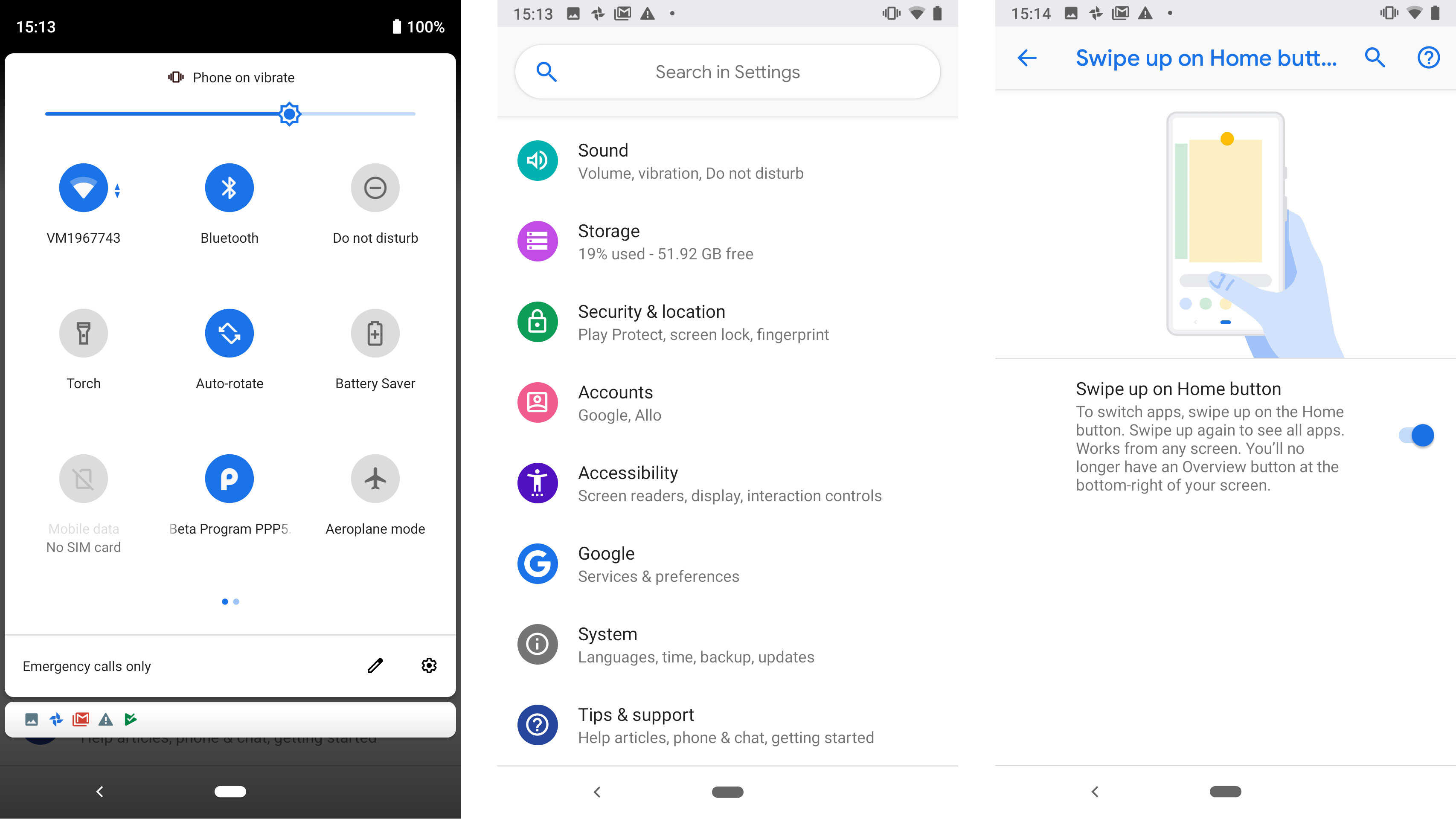The image displays three different smartphone screens side-by-side.

**Left Screen:**
The screen on the left depicts the quick settings menu of an Android device, accessible by swiping up from the bottom. The background is white, and the interface features a rounded rectangle design. At the top, a gray header states "Phone on vibrate." Below this, a progress bar is about three-fourths filled with blue, indicating the volume level, accompanied by a blue gear icon. Underneath the bar, a Wi-Fi symbol is displayed, indicating the network name "VM1967743." Next to this, a blue filled circle with a white Bluetooth icon is labeled "Bluetooth" in black. To its right, a light gray filled icon with a black circle and a line through it indicates "Do not disturb." At the bottom of the screen, in small black lettering, it says "Emergency calls only." To the right of this text is a pencil icon, slanted with the tip pointing towards the bottom left. Further right, a gear icon is shown for additional settings. Another bar below this features a series of icons from left to right: a gray image icon, a blue pinwheel icon, a red envelope icon for emails, a dark gray triangle with a white exclamation point, and finally, the Play Store icon.

**Middle Screen:**
The center screen presents a detailed list of settings options on a smartphone. The categories listed are: Sound, Storage, Security & Location, Accounts, Accessibility, Google, System, and Tips & Support.

**Right Screen:**
The rightmost screen has a light gray background with blue text at the top stating "Swipe up home BUTT..." next to three icons: a magnifying glass, a circle with a question mark inside, and an arrow pointing to the left. The exact purpose of these icons is not specified in the caption, but they appear to be related to navigation and help features on the device.